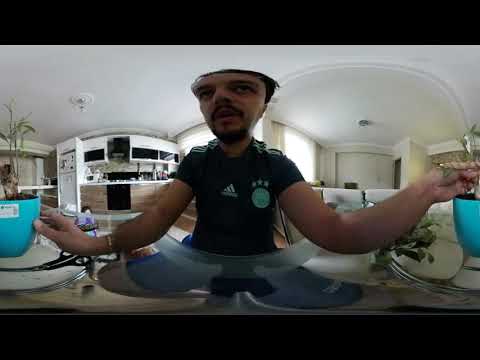The image is a 360-degree panoramic indoor setting showcasing a house with white walls and a white ceiling. At the center of the image, there's a man with short black hair, olive skin, a black beard, and a goatee. He is wearing a black short-sleeved Adidas shirt, featuring a white Adidas triangle logo, a green circular patch with three stars above it, and white stripes on the shoulders. The man is sitting behind a glass table, and his bottom half is obscured underneath it. He extends his arms to the sides, with each hand touching a blue flowerpot filled with dirt, containing growing plants or herbs. His elbows rest on the table, and there are scissors next to one of the pots.

In the background on the left side of the image, there is a kitchen area visible, including a refrigerator, cabinetry, and a sink. On the right side of the image, you can see a living room space with a couch. The top of the man's head appears slightly cut off due to the camera angle, and the curved ceiling is also visible towards the right side of the image. The man's face is subtly distorted into an upside-down triangular shape due to the panoramic lens effect.